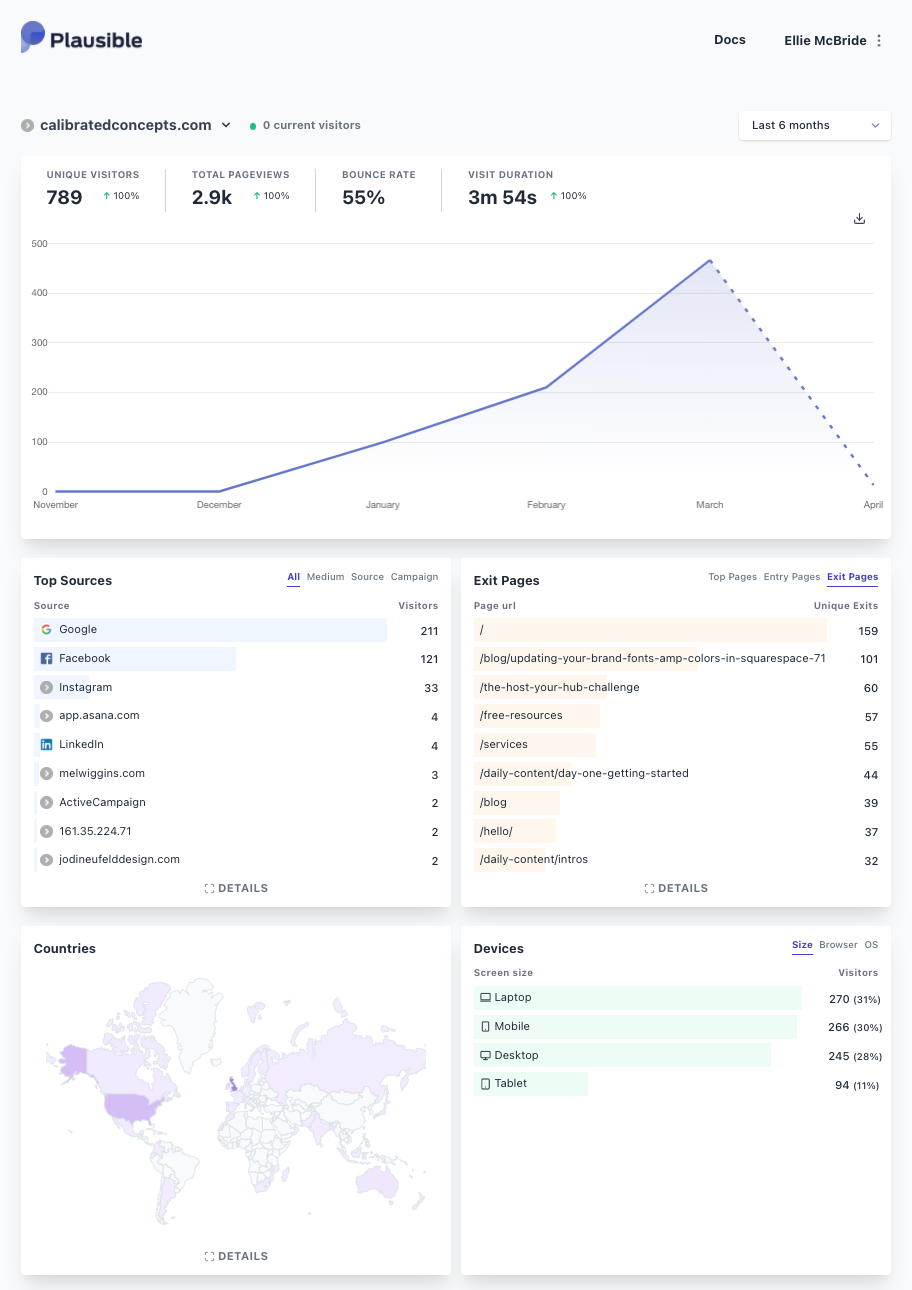A detailed caption for the image could be:

"Dashboard displaying web analytics for calibratedconcepts.com, logged in by L.E. McBride. The page is titled 'Plausible' at the top left, with 'Docs' on the right. The analytics cover a period from November to March, showing various statistics and graphs. Key metrics include 789 unique visitors, 2.9k total page views, a 55% bounce rate, and an average visit duration of 3 minutes and 54 seconds. The top sources of traffic are Google, Facebook, and Instagram. The most common exit page is the homepage (indicated by a forward slash). Geographic data shows the majority of visitors are from the U.S., with some activity from England. The device analysis indicates that laptops are the most commonly used to access the site."